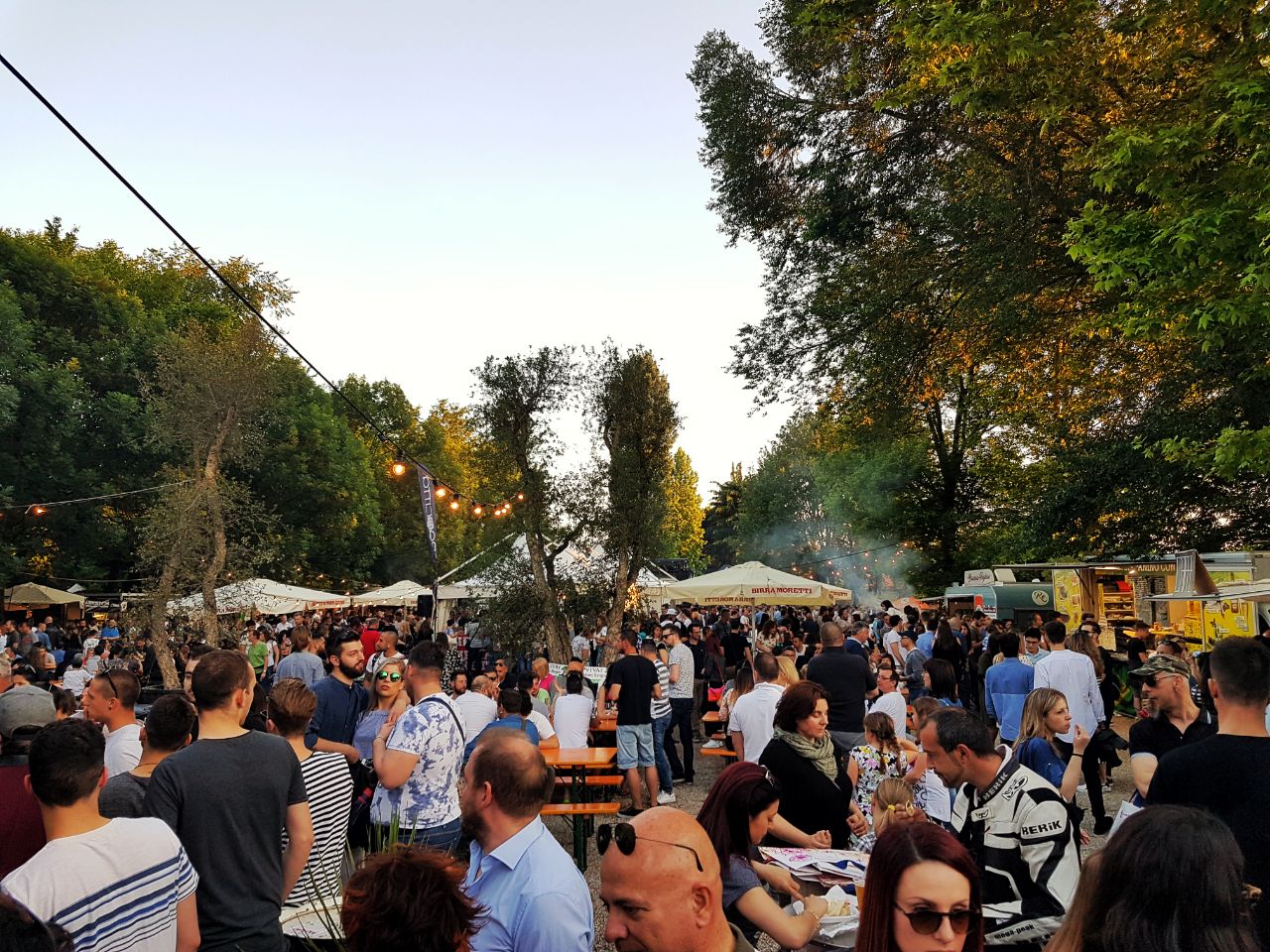The photo captures a bustling outdoor event, possibly a street fair or a festival, held during the early evening as the sky transitions to an almost gray hue, signaling the approaching night. The large crowd, easily numbering over a hundred participants, is the main focus, filling the foreground with a mix of seated and standing individuals. You can discern several yellow canopies of tents scattered among the people in the background, along with the presence of a yellow food truck on the far right. A wire hung with small illuminating lights extends from the top left to the distant background, casting a faint yellow glow. Smoke rises in the right background, likely from a barbecue or cooking activity. The setting is lush with trees; a prominent tree stands tall in the center back, and the left side is densely populated with foliage. People are dressed in warm-weather attire, with many in shorts and short sleeves, suggesting a pleasant evening temperature.